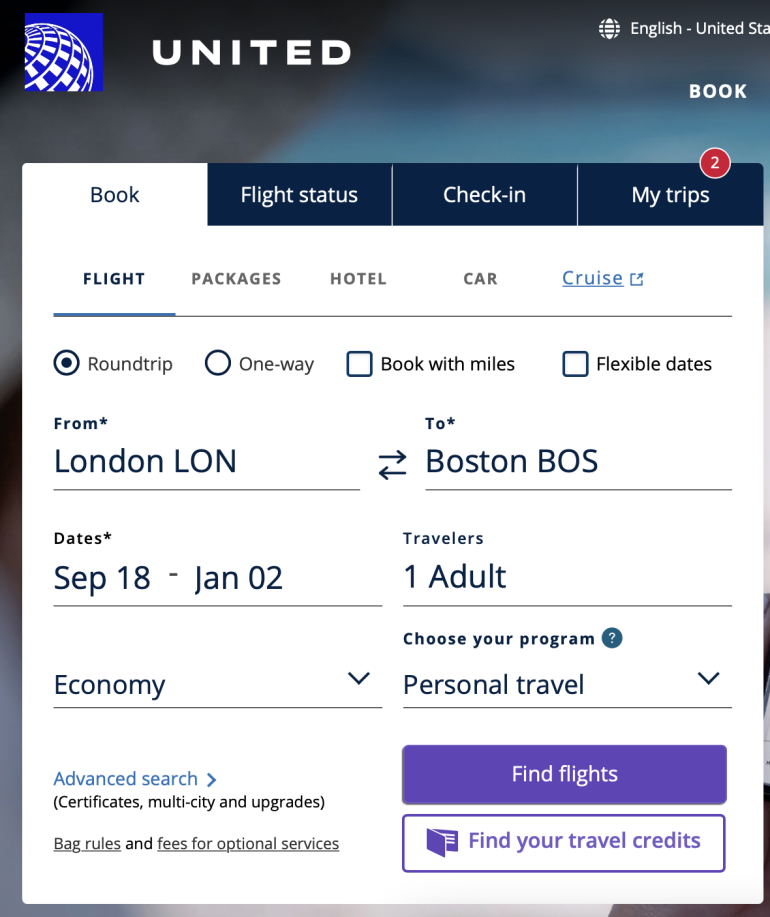Screenshot from United Airlines Flight Booking Website

This screenshot captures the United Airlines website interface for booking flights. At the top, the word “United” is prominently displayed. To its left is a small blue box that contains an icon resembling a globe, with text indicating the language setting: "English (United States)." On the right-hand side of the top bar, a white book icon is visible.

The main section shows the booking information for a roundtrip flight from London to Boston. The interface provides several navigational options including 'Flight Status,' 'Check-in,' and 'My Trips.' Notably, the 'My Trips' option features a small red circle with the number "2" inside, likely indicating pending actions or notifications.

Below these options are tabs for 'Flight,' 'Packages,' 'Hotel,' 'Car,' and 'Cruise,' with the 'Flight' tab currently selected. Further down, users can choose between booking options such as 'Roundtrip,' 'One-way,' 'Book with Miles,' and 'Flexible Dates.' The 'Roundtrip' button is currently selected, displaying details for a journey from London (LON) to Boston (BOS) with travel dates from September 18th to January 2nd. The traveler information indicates one adult in Economy class, classified under 'Personal Travel.'

Beneath these details is a prominent purple rectangular box labeled "Find Flights." Additional options include links for "Find Your Travel Credits" in purple and, to the left, options for "Advanced Search," "Certificates," "Multi-city," and "Upgrades."